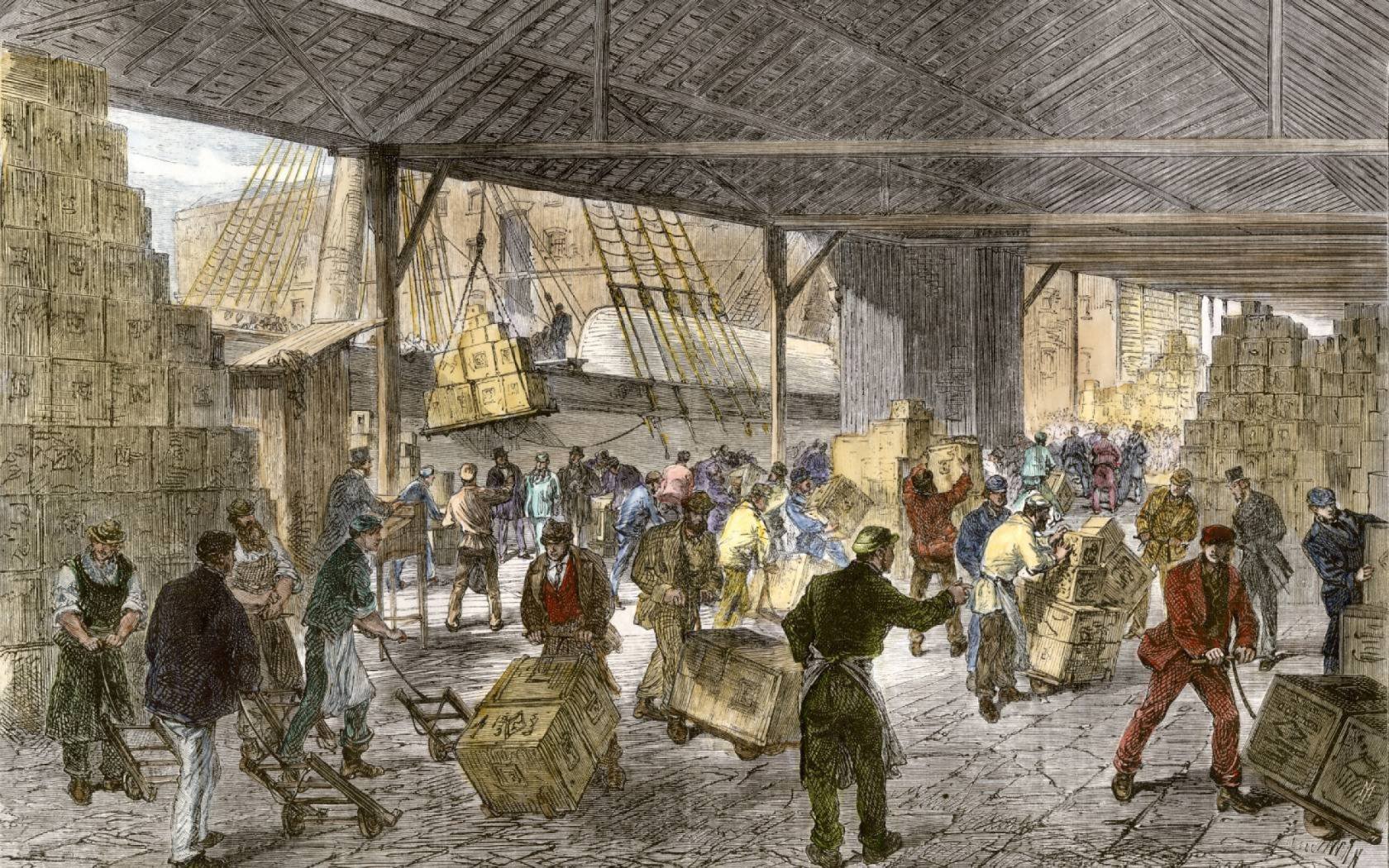The image is a detailed, hand-drawn depiction of a bustling early 20th-century dock scene. It features a roofed structure without walls, supported by columns, allowing a clear view of the activities inside. The floor is made of stone or gray tile pavers. At the center of the action are dozens of workers—some in suits, others in aprons—busily moving wooden boxes. They carry the boxes by hand, push them on carts, and stack them into towering piles scattered across the scene. A man stands prominently, delegating and pointing directions. In the background, to the left, a sail-powered cargo ship is visible, with a crane lowering boxes from the ship onto the dock. The colors in the drawing range from black, white, gray, and brown to mustard yellow, red, cranberry, and blue. This old, skillfully crafted drawing captures the industrious atmosphere of a port or harbor, with men diligently handling cargo under an expansive open-roof area.